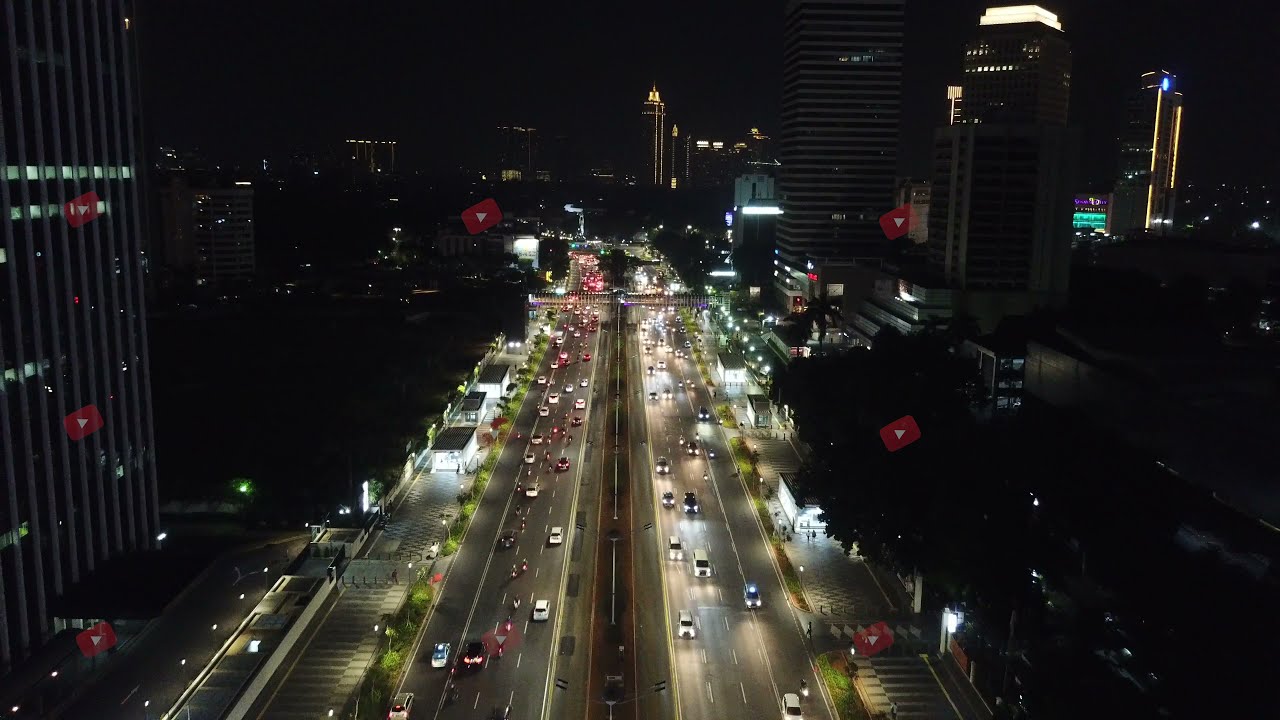This captivating aerial nighttime shot showcases a bustling highway threading through a vibrant metropolis. The road, possibly a broad divided highway with four lanes in each direction, is lined with a mix of small buildings and towering skyscrapers on both sides, their lights twinkling against the dark night sky. The central focus is the densely packed traffic, the headlights and streetlights illuminating the scene with a mesmerizing glow. Interspersed along the edges of the road are strikingly bright bus stops, adding to the urban tapestry. Unique to this image are several small, tilted, semi-transparent YouTube play button watermarks scattered across the scene, suggesting it might be a screenshot. Amidst the architectural giants and flowing traffic, the occasional pedestrian is visible, adding a touch of human presence against the backdrop of the city's grandeur.